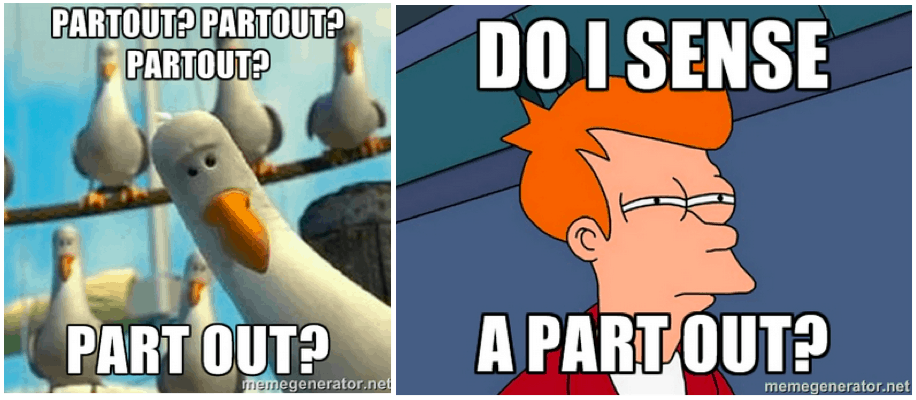This image features two side-by-side memes, both with cartoon drawings. The left meme showcases a light blue background, resembling a scene on a ship, where three seagulls are perched on a brown branch. Another seagull, with a bright orange beak, is positioned in the front corner, staring straight ahead. The top text in white letters reads "partoutpartoutpartout?", while the bottom text says "part out?" The right meme shows a cartoon character with short orange hair, squinting suspiciously to the side against a blue and green wall backdrop. The text above him reads, "Do I sense a part out?" A watermark on the bottom right corner indicates "meme generator.com." These memes, placed side by side and designed for humor, are likely intended for social media sharing.